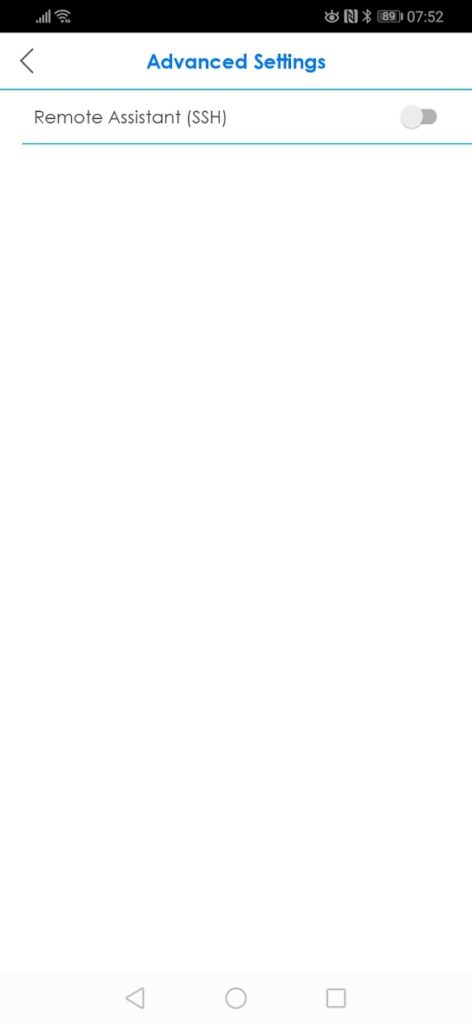The image showcases the top quarter of a smartphone screen. At the very top, a black status bar spans from left to right. On the left side of this bar, light gray icons represent cell signal strength; a series of ascending bars indicate coverage, accompanied by a curved signal icon. To the right, there are four distinct icons providing phone status information. One of these icons shows the number "89," likely indicating the percentage of battery remaining, followed by a small battery icon. Further right, the time is displayed as "07:52."

Beneath the black status bar is a gray arrow pointing left, situated on a white background. This background frames the heading "Advanced Settings" with both "A" and "S" capitalized. A light blue line underscores this heading, acting as a separator from the subsequent section.

The next section, also on a white background, begins with the title "Remote Assistant" with both "R" and "A" capitalized. To the right of this title, "SSH" is enclosed in parentheses. A gray oval toggle switch appears next to it, with the circle in the switch positioned to the left, indicating it is toggled off. Another blue line, teal in color, underscores this section.